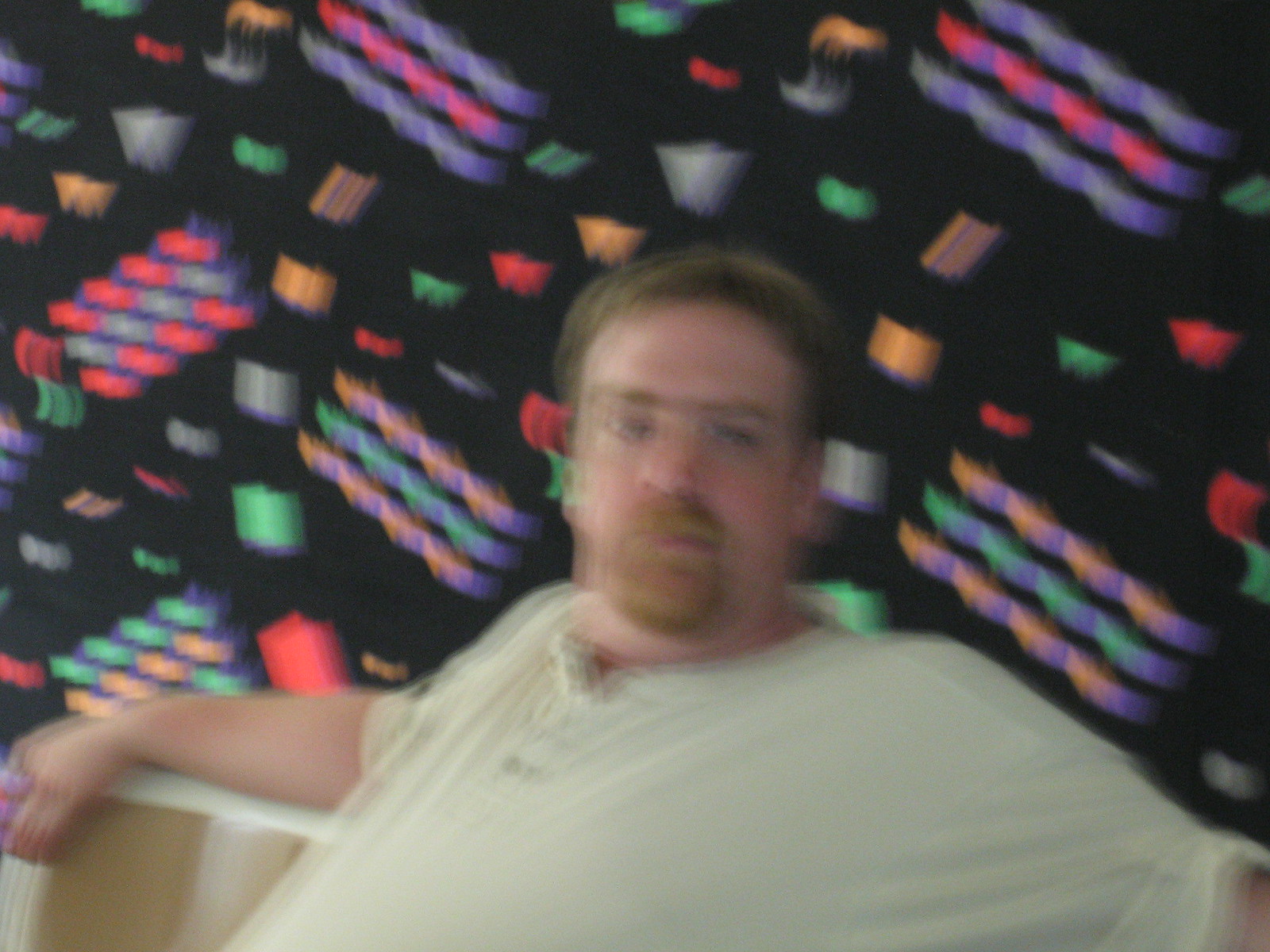The photograph captures a slightly blurry image of a Caucasian male with short brown hair, a brownish mustache, and a goatee. He is wearing a cream-colored shirt that features a few buttons at the neckline but does not button all the way down the front. It is unclear whether the shirt is short-sleeved or if the sleeves have been pushed or rolled up above his elbows. The man is facing towards the viewer, with a possible slight tilt of his gaze to the right. In the background, a black wall adorned with vibrant neon abstract designs in green, orange, purple, and pink creates a festive atmosphere reminiscent of confetti and ribbons. The man is seated on a piece of furniture, also in a creamy tan color, with his right arm casually draped over its back. Despite the photo's blurriness, these details provide a vivid portrayal of the scene.